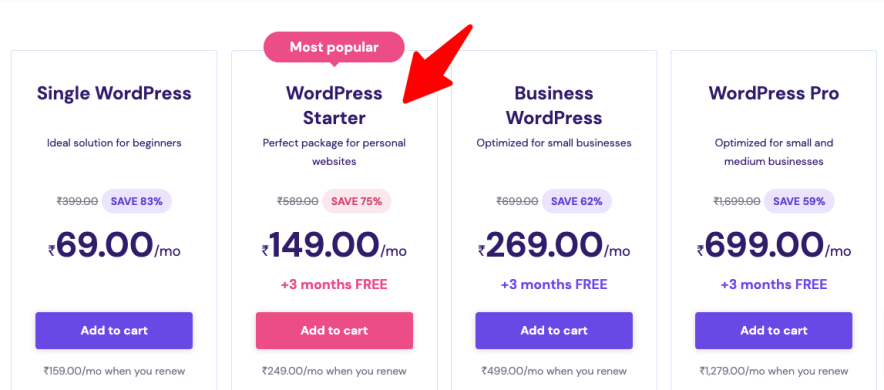This image displays a set of online package options for WordPress hosting, each tailored to different user needs and featuring significant discounts.

**Option 1: Single WordPress**
- **Description:** Ideal solution for beginners.
- **Original Price:** $3.99/month (strikethrough).
- **Discount:** Save 83%.
- **Current Price:** $0.69/month.
- **Action:** Add to cart.
- **Note:** An icon resembling lightning, likely indicating a currency symbol.

**Option 2: WordPress Starter (Most Popular)**
- **Description:** Perfect package for personal websites.
- **Original Price:** $5.89/month (strikethrough).
- **Discount:** Save 75%.
- **Current Price:** $1.49/month.
- **Bonus:** Additional 3 months free.
- **Action:** Add to cart.

**Option 3: Business WordPress**
- **Description:** Optimized for small businesses.
- **Original Price:** $6.99/month (strikethrough).
- **Discount:** Save 62%.
- **Current Price:** $2.69/month.
- **Bonus:** Additional 3 months free.
- **Action:** Add to cart.

**Option 4: WordPress Pro**
- **Description:** Optimized for small and medium businesses.
- **Original Price:** $16.99/month (strikethrough).
- **Discount:** Save 59%.
- **Current Price:** $6.99/month.
- **Bonus:** Additional 6 months free.
- **Action:** Add to cart.

Each option is succinctly presented with both its original and discounted price, along with any additional promotional offers, encouraging users to take action by adding the packages to their cart.